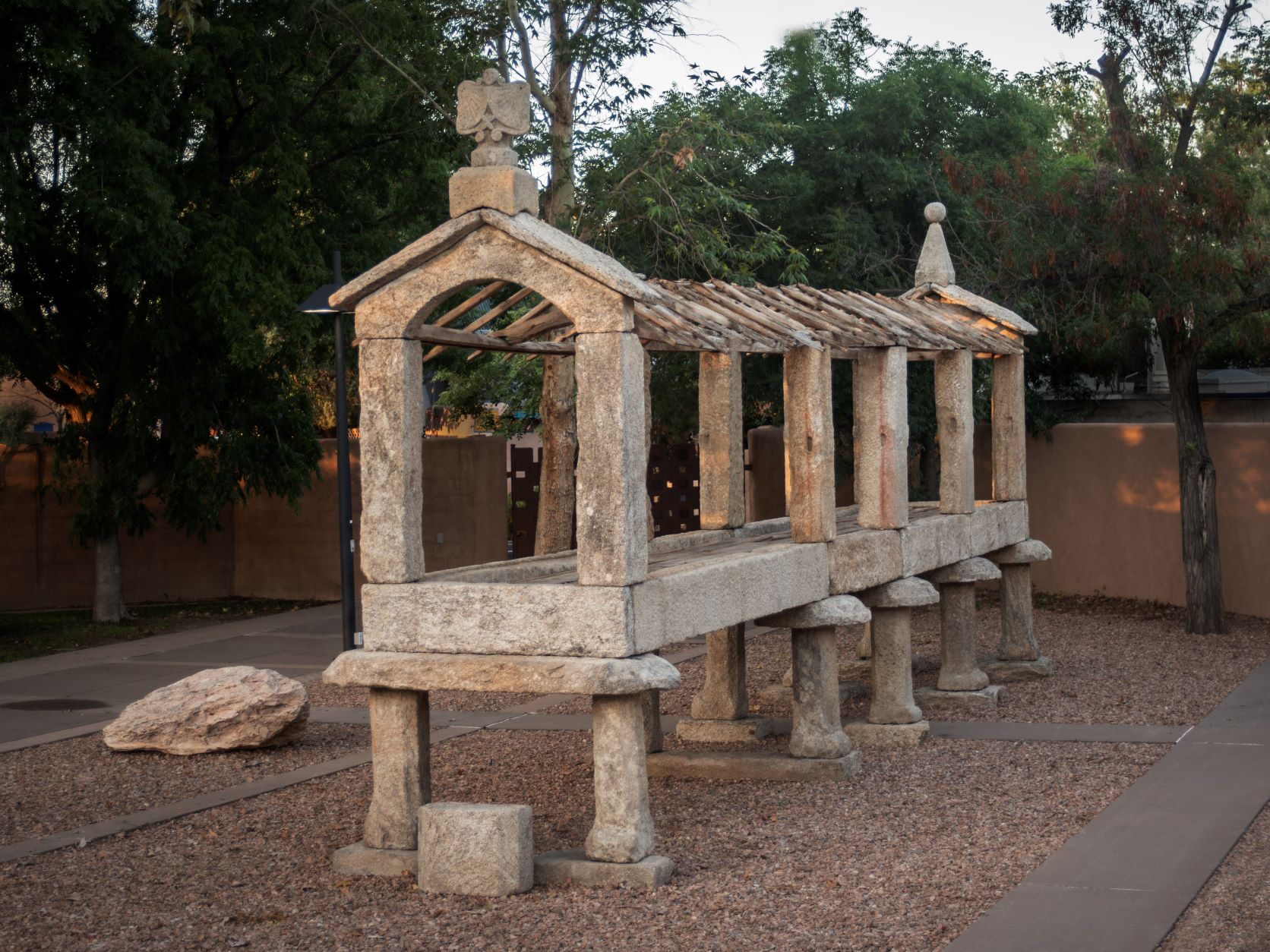The image depicts an outdoor stone structure resembling a small-scale, old church or elongated house, prominently displayed in a park-like setting. The structure is composed of five pairs of vertical concrete brick columns. These columns support a lengthy, open framework, which forms a tunnel-like shape. The roof of this structure consists of slanted stone slabs, extending from the front to the back. On top of these slanted stones are two distinct objects: one appears to be bird-like at the front, and the other is a triangle with a ball on top at the rear. The surrounding area is enclosed by a brick or brown fence, and there are trees lining the backdrop under a white, cloudy sky. The ground around the structure features stone walkways interspersed with tiny pebbles, creating paths for visitors to navigate through the serene, scenic environment.